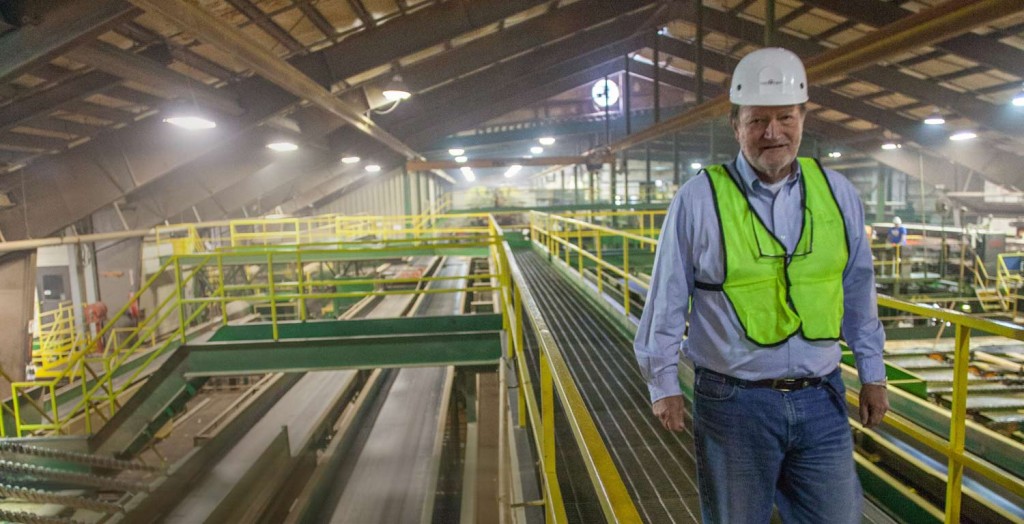In this detailed photograph taken inside an industrial factory, an older Caucasian man stands prominently on a catwalk, appearing to be the focal point of the image. He exudes a sense of happiness, with his glasses hanging around his neck and his mouth open as if he's talking. The man is dressed in a white hard hat, a vibrant lime green safety vest, a light blue button-up collared long-sleeve shirt, blue jeans, and a black belt. He stands on a non-skid tread catwalk, which has a dark green color, with surrounding yellow metal safety railings to prevent falls.

The factory setting includes a complex network of upper walkways and green staircases, supported by crisscrossing beams and metalwork visible on the steel roof above. The roof has sloped sections going to the left and right, and is brown with many pipes running across it. Below the catwalk, there are empty conveyor belts. In addition to the main subject, there is another person in the background on the lower level, also wearing a white hard hat and a blue t-shirt. The image captures the intricate industrial environment with precision and detail.